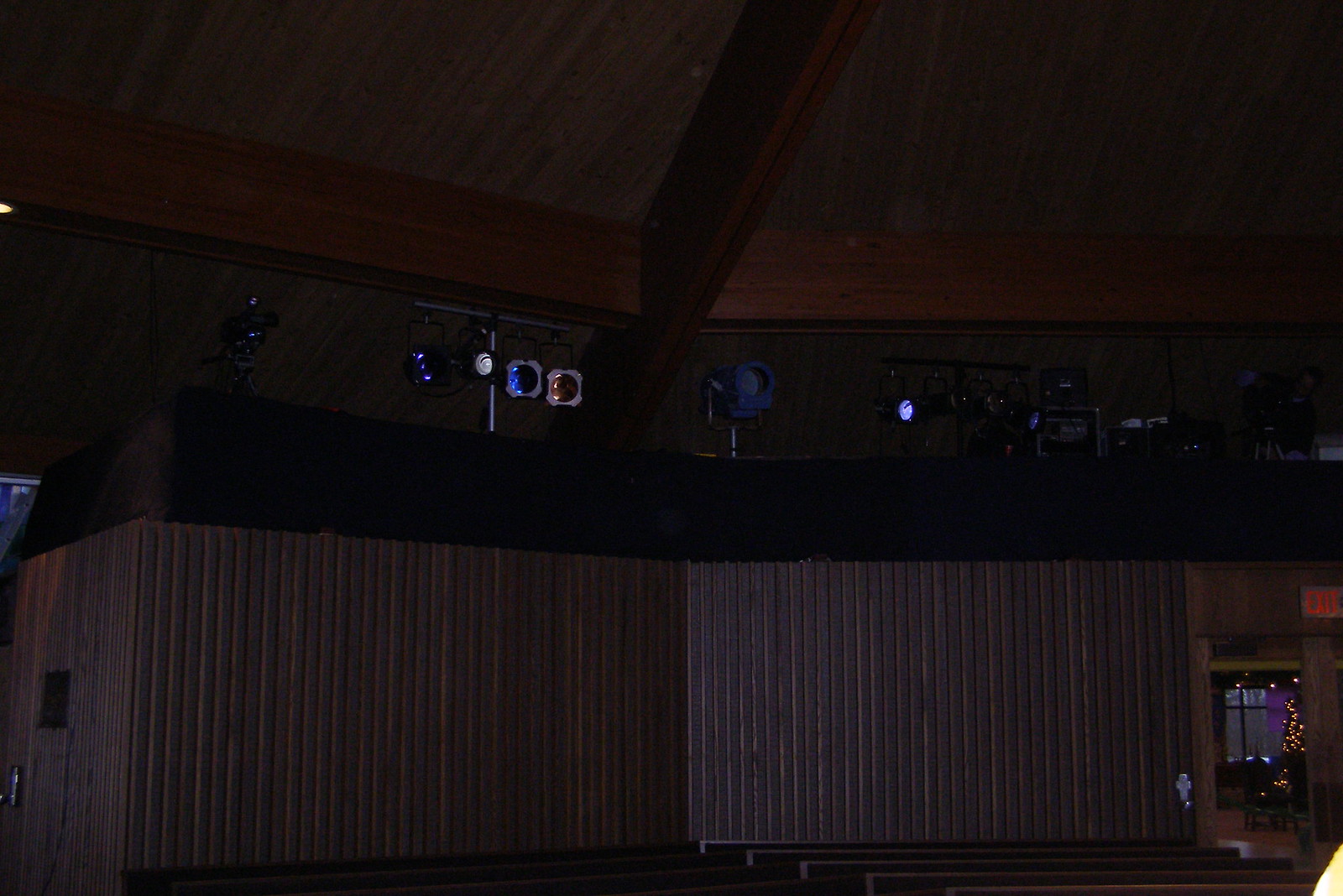In this extremely dark, nighttime color photograph, a dimly lit, rectangular, wooden structure dominates the lower third of the image. Though difficult to discern, it likely represents the side of a building, supported by the visible doorway in the bottom right corner which is adorned with a red-lit exit sign. Adjacent to this area appears to be a window. The structure could be interpreted as an interior space, possibly of a church, evidenced by the high, dark brown wooden roofing and beams extending across the top half of the photo, along with light fixtures reminiscent of stage lights. Above the structure, the image reveals various small lights—some gold, one blue, and others yellowish—possibly from a Christmas tree, enhancing the sense of an indoor, festively decorated setting.